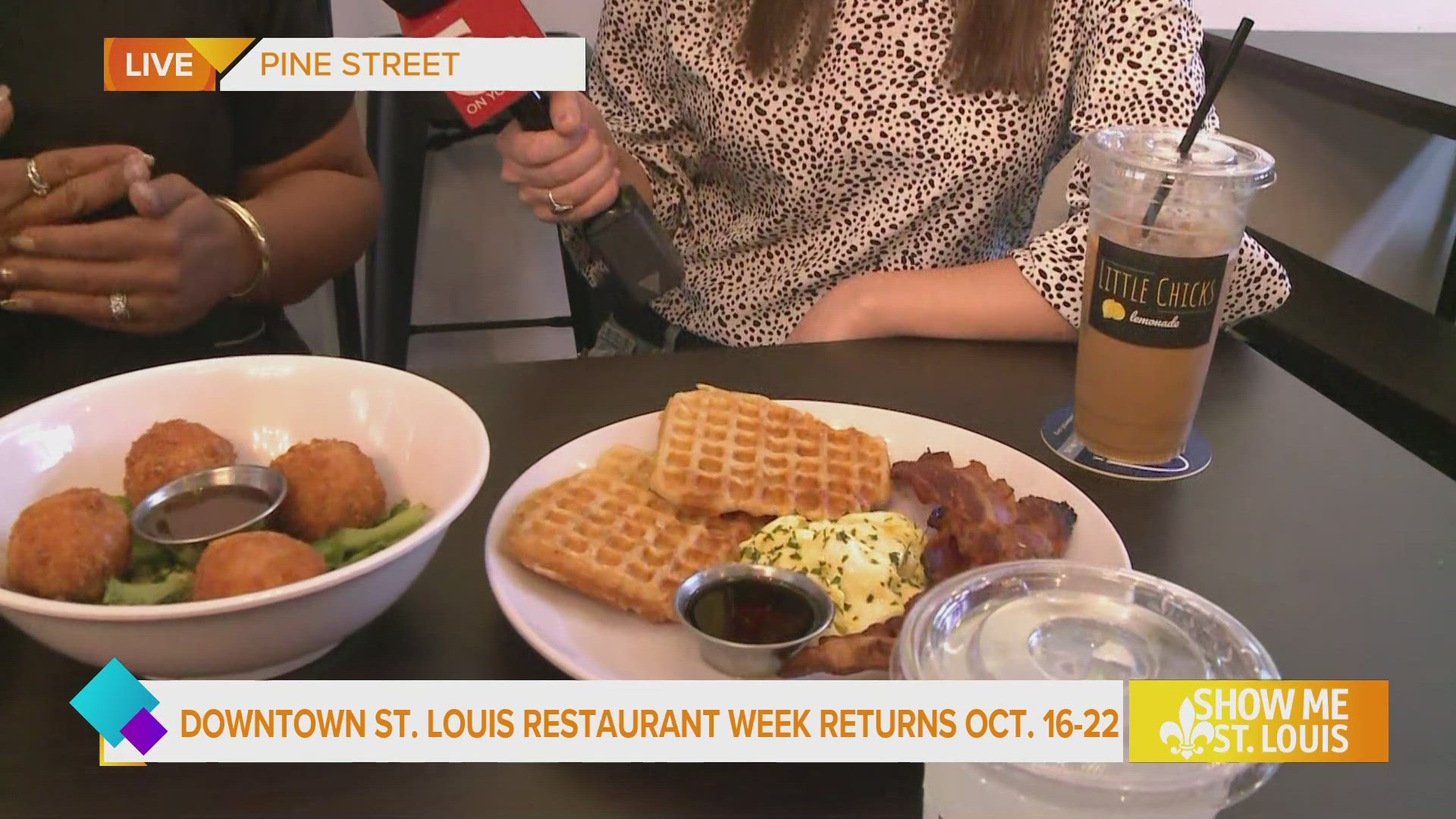The image is a vibrant advertisement, likely a screenshot from a TV or digital show, promoting Downtown St. Louis Restaurant Week, scheduled for October 16th to the 22nd. In the upper-left corner, there is a band with "Live" in white letters on an orange background and "Pine Street" in orange letters on a white background. Centered below this, two women are seated behind a grey table, engaged in conversation. The woman on the left, partially visible, is wearing a black short-sleeved shirt and has a gold bracelet, rings, and long nails. The woman on the right, with brown hair visible over her chest, is dressed in a white blouse adorned with red and dark dots and holds a microphone towards her companion.

The table in front of them features an array of food and drink items. To the left, a white bowl contains four golden-brown fried balls, likely doughnuts, with a small jar of sauce in the middle. Adjacent is a white plate holding two square waffles topped with bacon, a poached egg, and green sprinkles. Below the plate, a round silver container appears to hold more sauce. A plastic cup with a black straw and a sticker labeled "Little Chicks" stands out among the items, along with the visible top of another plastic cup.

Spanning across the bottom of the image is a large, white horizontal rectangle with orange text announcing, "Downtown St. Louis Restaurant Week returns October 16th to the 22nd," alongside the "Show Me St. Louis" logo, set against a yellow and orange gradient background. In the background, a stool and some shelves add to the setting’s ambiance, enhancing the overall promotional appeal of the image.